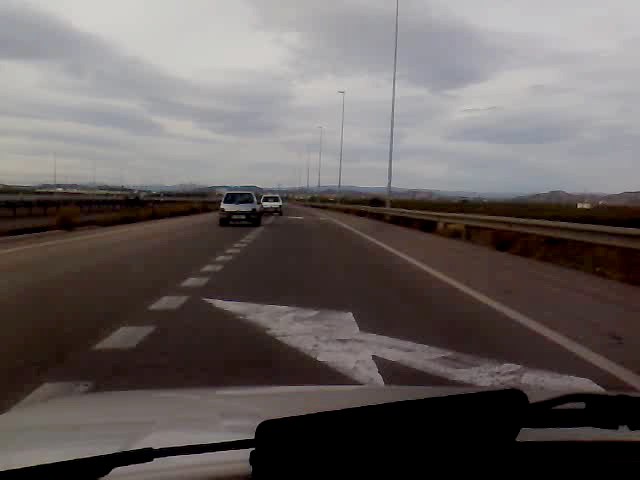This photograph captures the perspective from the driver's side of a moving silver car, likely suggesting it was taken while driving. The image includes a view of the car's hood and its black windshield wiper blades. Positioned in the far right lane, the car appears to be in the process of merging into an adjacent lane due to the visible white arrow on the road, signaling the lane's imminent end. Another similar arrow is seen further ahead. The scene also features a dashed white line marking the lane boundary that the car needs to cross. Two white vehicles occupy the lane the car is aiming to merge into. Guardrails, painted silver, line both sides of the road, adding a sense of safety and direction. Streetlights are spaced along the roadway, extending towards the horizon, providing a guide for the route ahead.